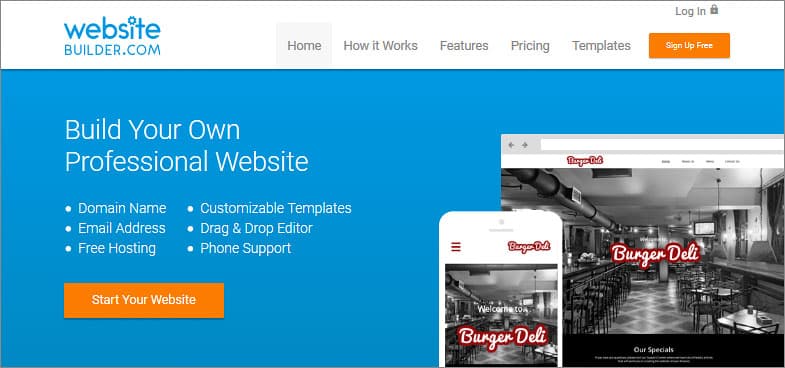This is a detailed screenshot of the homepage of WebsiteBuilder.com. The main focus of the webpage is a prominent blue box positioned towards the lower center, containing an advertisement for the company's services. The blue box features white text that provides information on the key offerings of the platform.

On the left-hand side, in white text, there is a call to action that reads, "Build your own professional website." This section elaborates on the benefits provided, such as domain name hosting, email addresses, and phone support.

In the bottom left corner, an orange box with white text prompts users to "Start Your Website." Clicking this button redirects users to another page where they can enter details and begin creating their website.

The bottom right section features an example of a website created using the platform, showcasing an enticing "Burger Deli" theme. This section includes images of both a mobile phone and a computer screen, demonstrating the platform's capability to create websites that are optimized for both mobile and desktop views.

At the top of the screenshot, a white horizontal navigation bar contains links labeled "Home," "How It Works," "Features," and more, offering a gateway to different sections of the website for further information on building a website with this company.

The logo and name of the website, "WebsiteBuilder.com," are prominently displayed in blue text in the top left corner. On the top right, there's another orange box with white text that says "Sign Up Free," which directs users to a sign-up page to start building their own website.

This detailed layout and design effectively guide users through the initial stages of website creation, providing clear navigation and relevant information on the services offered.